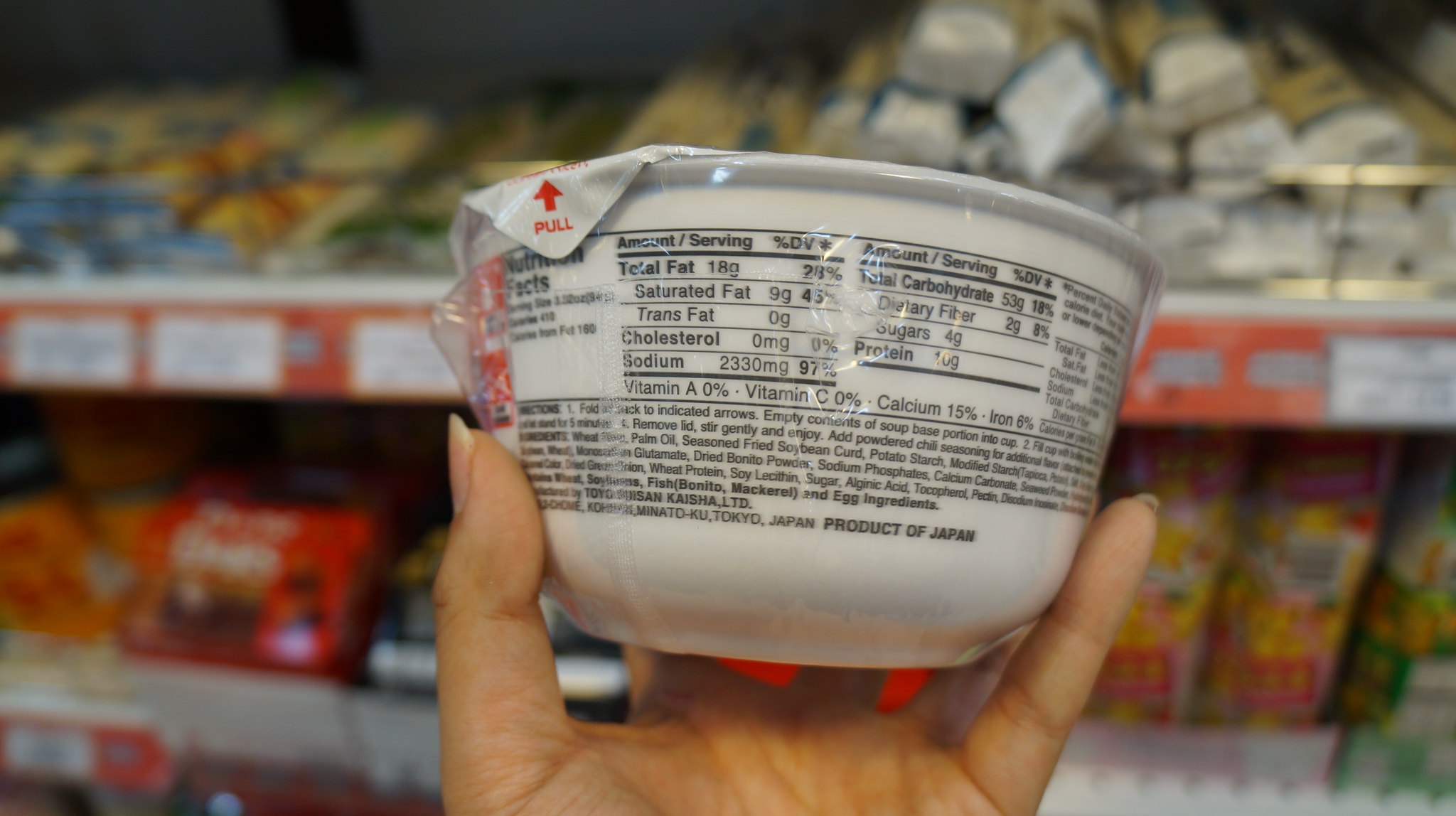A close-up photograph captures a left hand holding a white plastic bowl, enveloped in clear plastic wrap, and sealed with a plastic or aluminum cover. This cover features a prominent red arrow labeled "Pull." The hand, with its delicate, medium-length fingernails, appears to belong to a woman. 

The background, though blurred, suggests the setting is near two shelves stocked with various food items. Visible on the bowl is a detailed label containing nutrition facts: "Total Fat: 18 grams," "Cholesterol: None," "Sodium," and "Total Carbohydrates." Additionally, there are instructions stating, "Fold here," along with two indicated arrows and directions to "Empty contents of soup base," likely to portion it into cups before making the soup.

The ingredients list includes items such as wheat, palm oil, seasoned fried soybean curd, potato starch, and modified starch, among other components. The label at the bottom of the bowl reads "Product of Japan," indicating its origin.